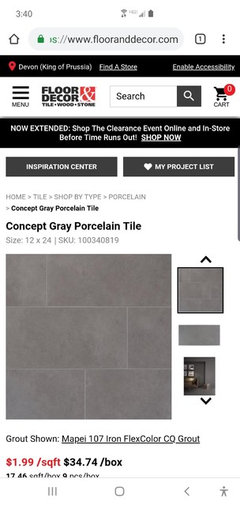This image is a screenshot taken from the FloorandDecor.com website displayed on a smartphone. The screenshot is in a portrait orientation typical of a phone display. At the top of the screen, it shows a location pin icon next to the text "Devon King of Pressa" with an option to "find a store" and a prompt to "enable accessibility."

Below, there's a navigation menu symbolized by three horizontal black lines. To the right of it is the "Floor and Decor Tile, Wood, and Stone" logo, followed by a search bar and a cart icon indicating that it is currently empty with a red circle showing "0" items.

Scrolling down, there’s a prominent black rectangle banner that reads "Now Extended, Shop the Clearance Event Online and In-Store Before Time Runs Out," accompanied by a "Shop Now" link underlined for emphasis. 

Further down, there is an "Inspiration Center" section highlighted in gray. Towards the right, there's a heart icon labeled "My Project List." 

The detailed content shows someone viewing a product: "Concept Gray Porcelain Tile." It is specified as "Size 12 x 22" and displays its SKU number. The pricing information is highlighted in red, indicating "$1.99 per square foot" and "$34.74 per box."